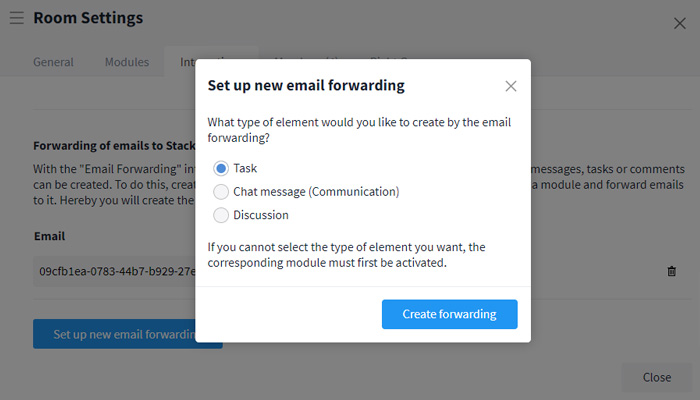**Caption:**

The screenshot displays a user interface with a white background that has a grayish haze due to a central pop-up window. 

**Background Elements:**
- In the top-left corner, there are three horizontal black lines stacked vertically. To the right, the bold text "Room Settings" is displayed. On the far right, there's a black "X".

**Tabs and Menu Options:**
- Below "Room Settings," there are three tabs:
  1. The first tab, labeled "General," is in black.
  2. The second tab is labeled "INT" and extends under the pop-up window.
  3. Below these tabs is bold black text reading "Forwarding of Emails to Stack," which also extends under the pop-up window. This line has three black lines coming from the left side, with two lines extending to the right.

**Input Fields and Action Items:**
- Under these sections:
  - A bold black label "Email" appears above a rectangular field filled with numbers.
  - On the right side of this rectangle is a trash icon.
  - In the bottom left corner, a blue tab partially visible under the pop-up reads "Set up new email forward" in white text.

**Pop-Up Window:**
- The pop-up window features:
  - At the top-left corner of the pop-up, bold black text states "Set up new email forwarding."
  - On the top-right corner, there is a gray "X."
  - Beneath the title, small black text reads, "What type of element would you like to create by the email forwarding?"
  - Below this text, there are three circles outlined in gray:
    - The top circle is blue and labeled "Task."
    - The bottom two circles are gray, labeled "Chat Message" and "Discussion" respectively.
  - A note in black states, "If you cannot select the type of element you want, the corresponding module must first be activated."

**Primary Actions:**
- At the bottom right, a blue button with white text reads "Create Forwarding."
- A gray "Close" button is located on the bottom right of the pop-up.

This detailed caption should comprehensively describe the provided image.